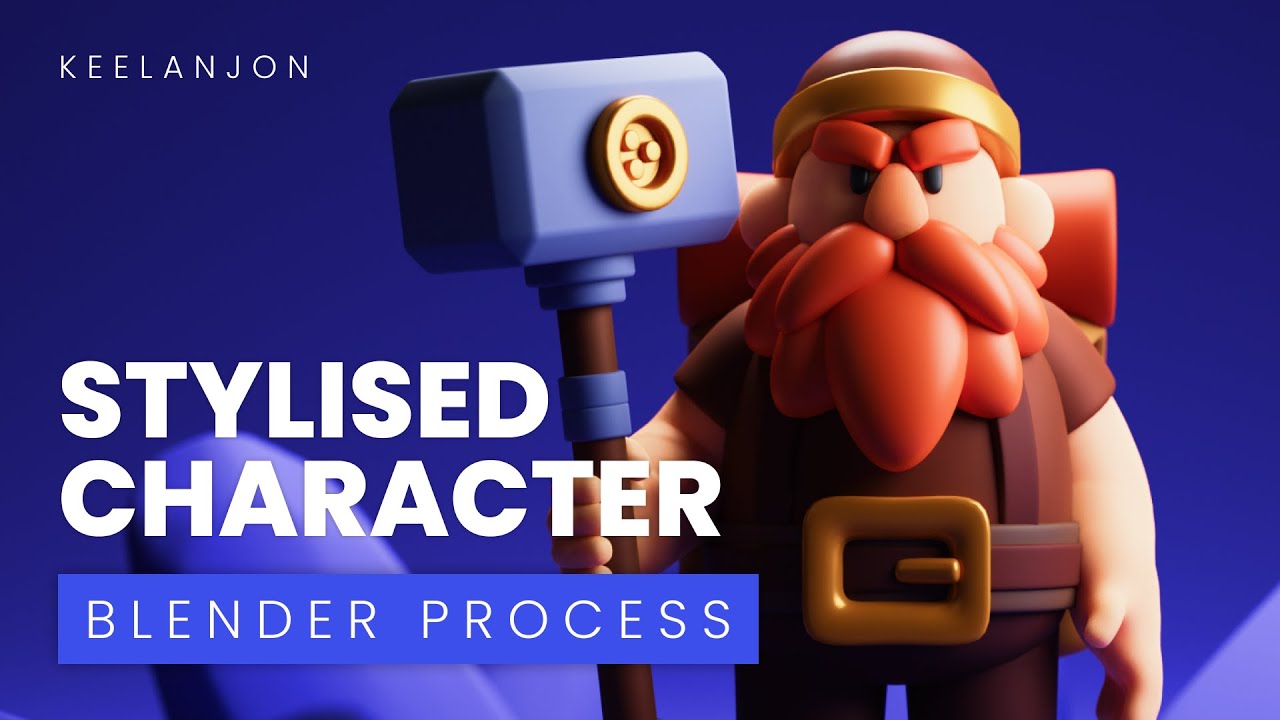The YouTube thumbnail showcases the artistry of creating stylized characters in Blender by Keelan John. Dominating the image is a highly detailed, semi-claymation figure resembling a dwarf gnome with striking features: a red, bushy beard and mustache, and thick, bushy eyebrows. He exudes a Norse aesthetic with an expressive, angry face, a bulbous nose, and a sturdy brown belt. The character is armed with an elaborate mallet, featuring a brown wooden handle adorned with blue rings and a bluish head with a gold circle. Additionally, he carries a backpack and wears a cap. The text "Keelan John" is prominently displayed on the top left, while "Stylized Character Blender Process" resides in the bottom left corner. The background is a textured, deep navy blue fading to indigo, adding depth and focus to the character, who appears to look directly at the audience, making it clear this thumbnail is designed for individuals interested in character modeling tutorials in Blender.